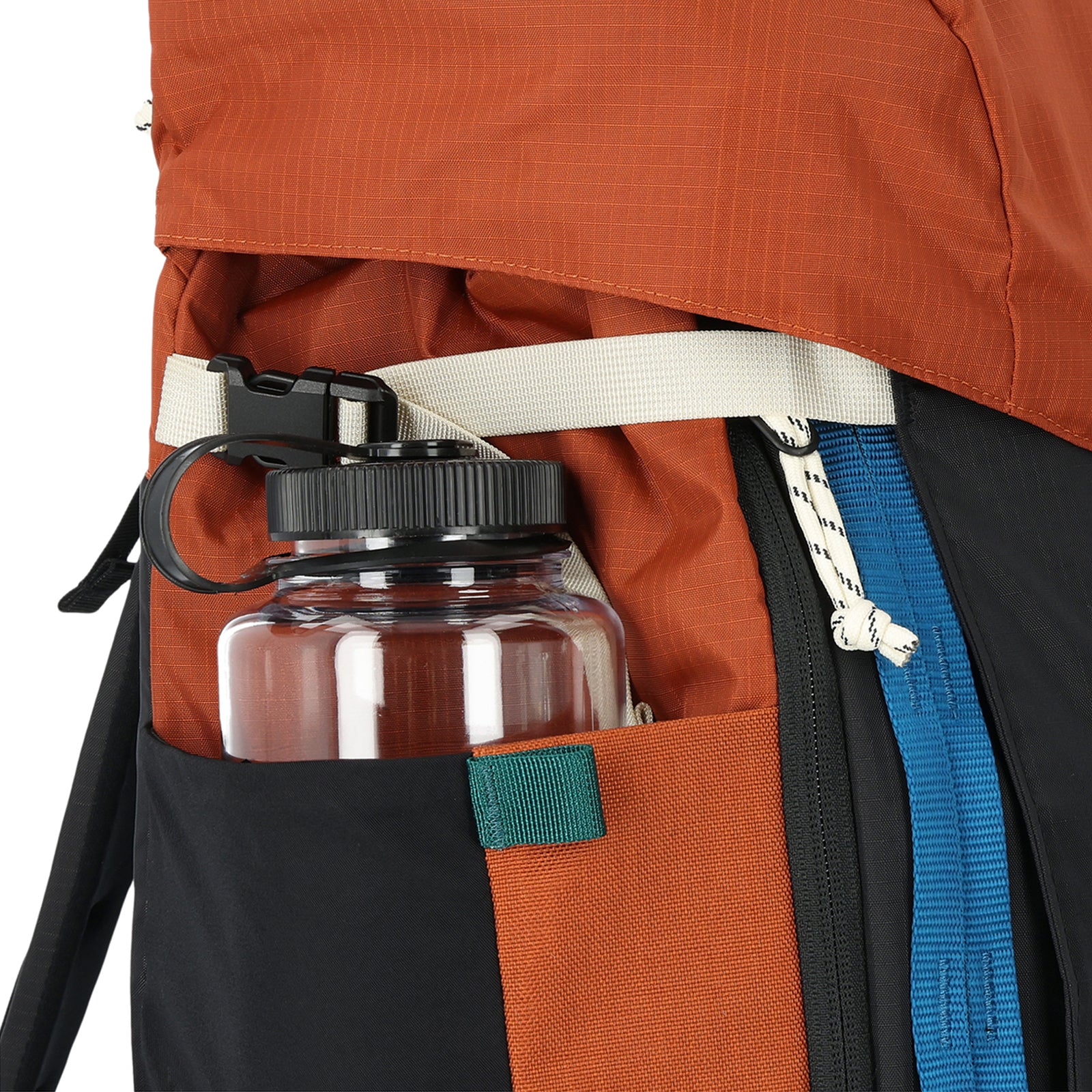This close-up shot captures a clear plastic water bottle with a black twist top and mouthpiece, securely nestled in an athletic short's generously-sized side pocket. The shorts feature a striking color combination of black and rust-red, further accented by a teal tab at the junction of these colors. The water bottle is firmly held in place by a black carabiner-type clip attached to white straps, adding both functionality and visual interest. Just beneath the pocket hem, a green loop can be seen, possibly for attaching additional gear. The person's shirt matches the rust-red color of the shorts, extending the cohesive color scheme. Additionally, a blue stripe and a black fabric detail are present near the bottle pocket, contributing to the overall intricate design of the athletic outfit.